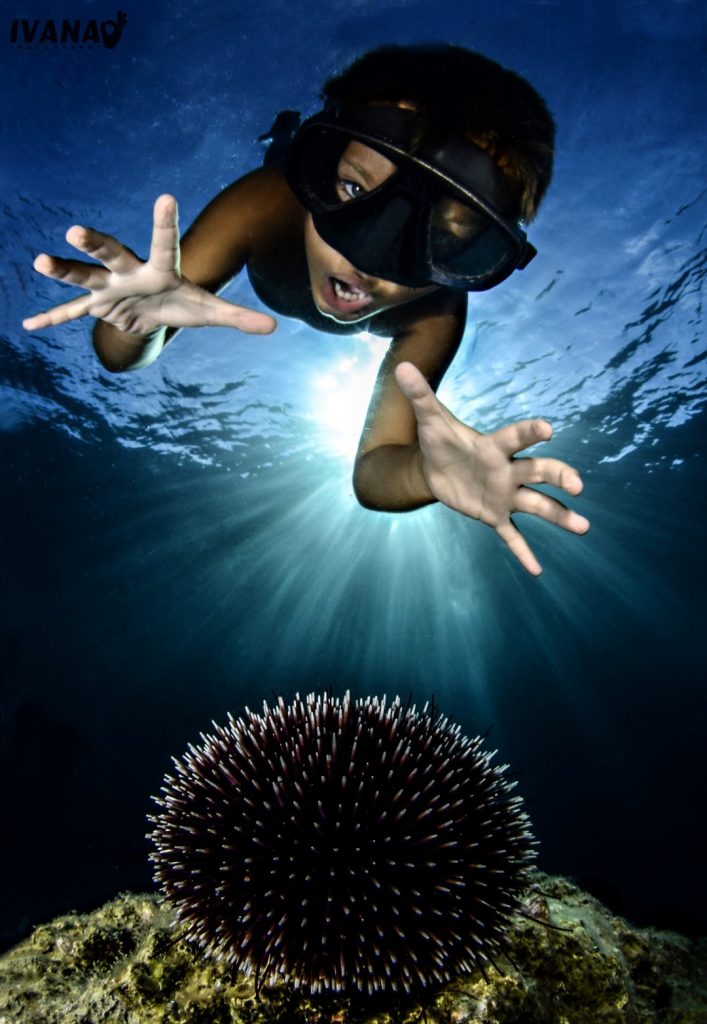In this high-resolution, portrait-mode underwater photograph, a child with a darker skin tone, approximately 10 years old, swims toward a sea urchin resting on a moss-covered rock in the foreground. The child, wearing black swimming goggles and scuba equipment, extends one hand towards the spiky black sea urchin but looks directly at the viewer with an open mouth, almost as if saying "blah". Illuminated by sunlight filtering through the clear blue water from above, the scene captures the vibrant and intriguing interactions beneath the ocean's surface, framed by shimmering sun rays in the background.